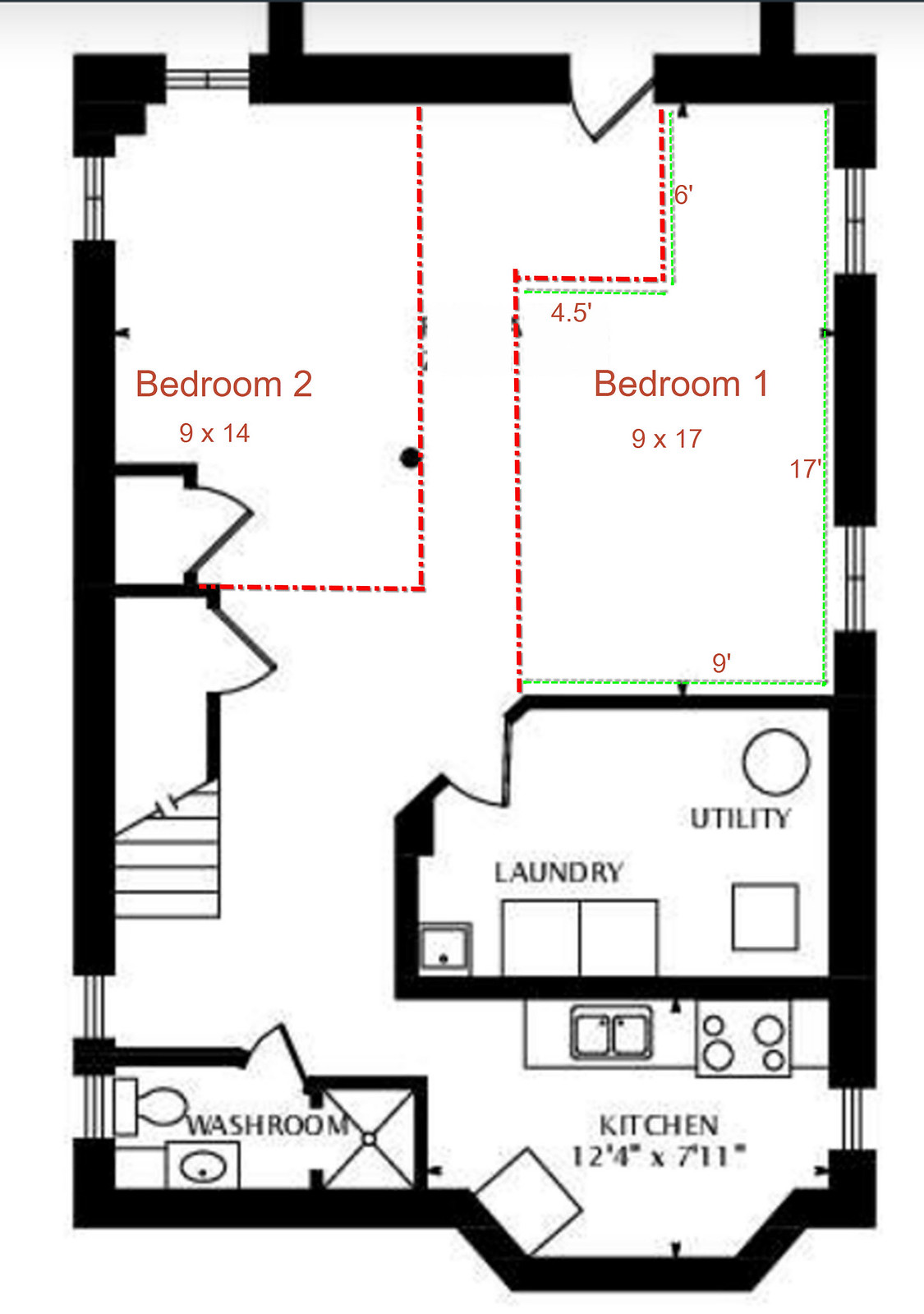This detailed floor plan depicts a rectangular building layout. Positioned in the lower right section of the rectangle is a 12.4 by 7.11 feet kitchen, which features a distinctive window that protrudes from the main rectangular wall. Directly to the left of the kitchen is a conveniently located washroom. Moving further upward and still to the right side of the layout, one encounters the laundry and utility room—essential for household maintenance and chores.

In the upper segments of the floor plan, two bedrooms are marked in red text. Bedroom One is situated in the upper right corner and measures 9 by 14 feet, providing ample space for a comfortable sleeping area. Bedroom Two, slightly larger at 9 by 17 feet, occupies the upper left corner, offering more room for additional furnishings or personal activities. These spatial arrangements and detailed dimensions provide a comprehensive understanding of the building's layout, ensuring clarity on the design and functionality of each room.